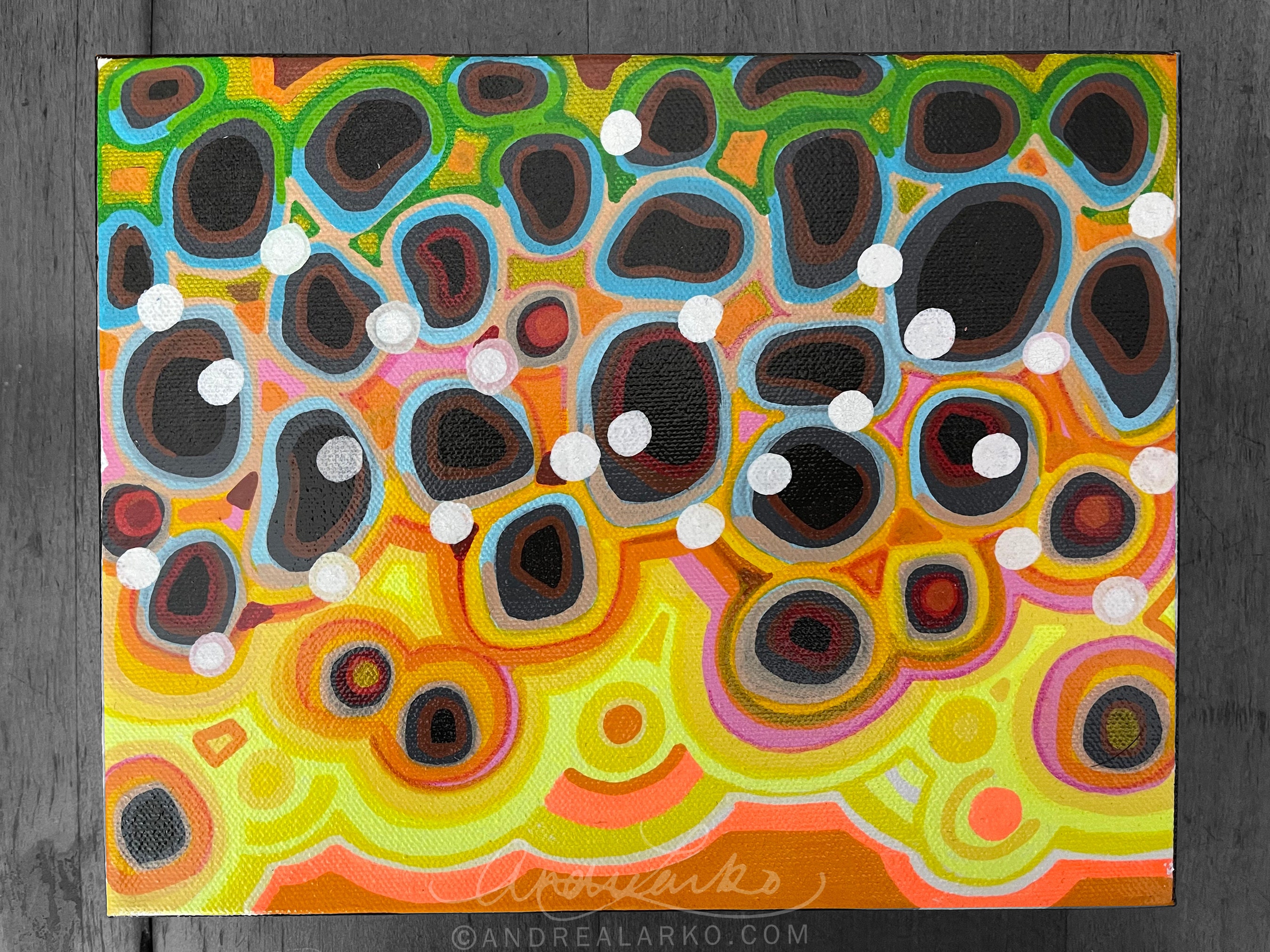The artwork is an abstract piece featuring a vivid collection of circular or splotch-like forms arranged on a background dominated by yellow and orange hues. The circles, primarily dark in the middle, are surrounded by varied color outlines—mainly blue, gray, and brown. The composition transitions from predominantly orange and yellow at the bottom to greener and bluer tones as you move upwards. Among the black spots scattered across the piece, there are approximately 25 smaller white spots that are more concentrated towards the top. The painting is framed in dark gray wood and features the artist's name, "AndreLarco," at the bottom, though it is not easily legible. Additionally, there is a web address, 'AndreLarco.com', inscribed at the bottom of the frame.